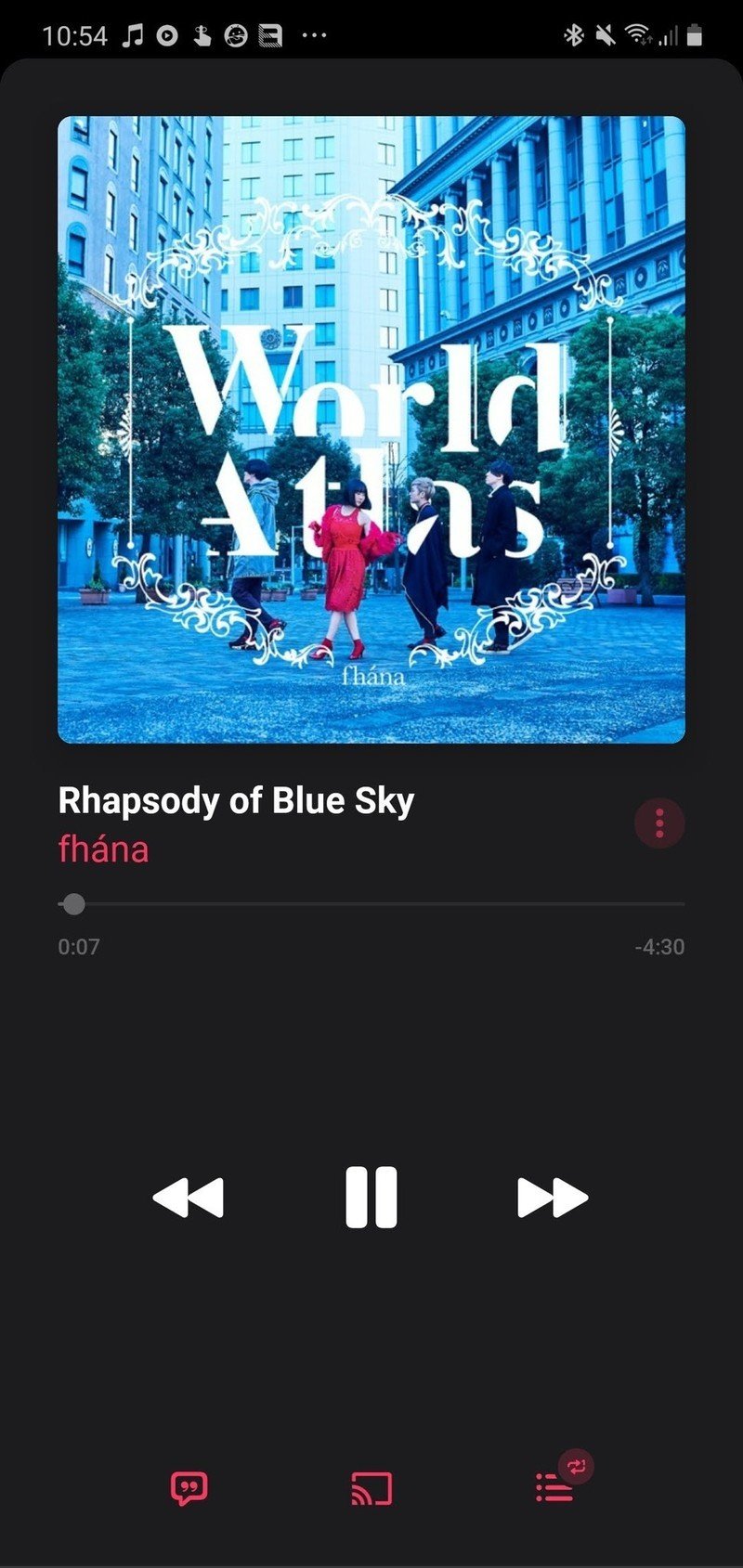An image depicting a music app interface on a smartphone with a black background. The status bar at the top shows the time as 10:54, followed by icons for music, play, and several other symbols including a pointer finger, a cat, and a buckle. On the right side of the status bar, there are indicators for Bluetooth, audio muted, Wi-Fi, and battery level.

Directly below the status bar is the album cover for "World Atlas" by FHANA, depicting the album art prominently. Below the album cover, the song title "Rhapsody of Blue Sky" is displayed with the band name, FHANA, highlighted in red. The playback time shows that 7 seconds of the song have been played out of a total duration of 4 minutes and 30 seconds. Beneath the playback time are the control buttons for play, rewind, and forward.

At the bottom of the screen, there are three icons in red – quotation marks, screen share, and a menu icon with three dots, offering additional options for the user.